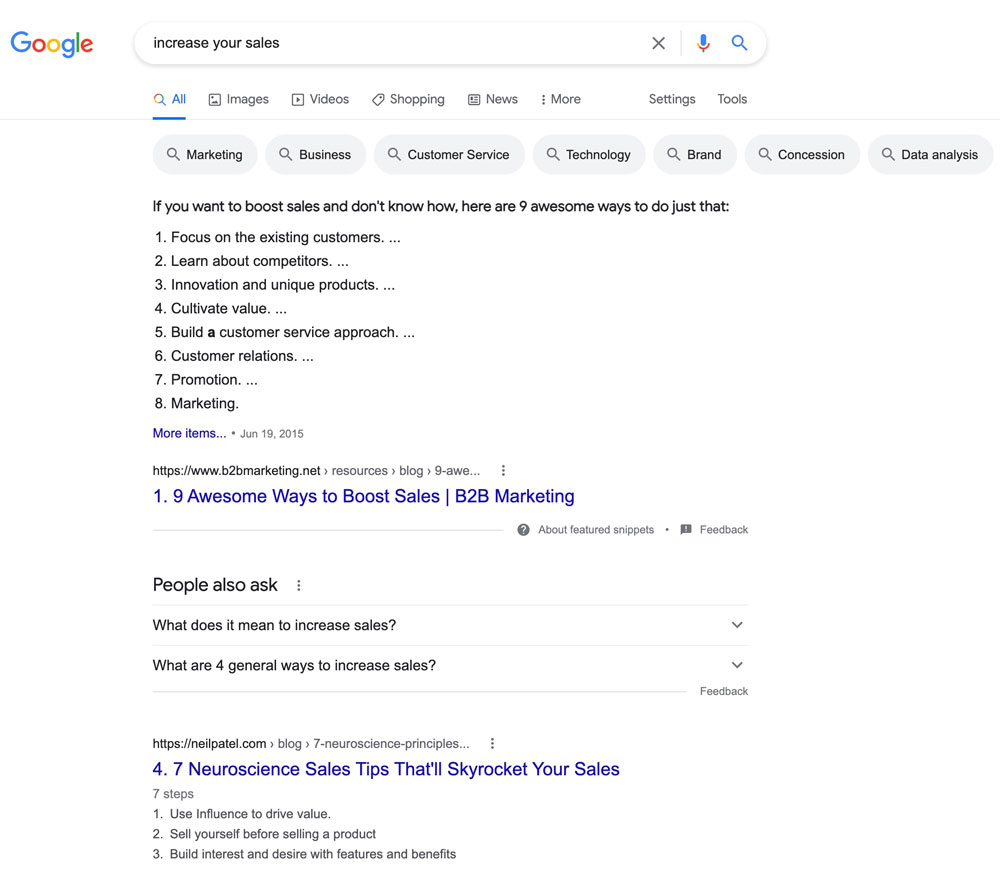In this image of a Google search results page, the background is predominantly white. In the upper left corner, the iconic Google logo is displayed in its traditional colors: blue, red, yellow, and green. To the right of the logo is a search bar with the query "increase your sales" inputted. Adjacent to the search bar, on the right, are the microphone and magnifying glass (search) icons.

Below the search bar, a row of tabs is visible, offering options such as "All," "Images," "Videos," "Shopping," "News," "More," "Settings," and "Tools." Underneath these tabs, there are several light gray bubbles featuring categories like "marketing," "business," "customer service," "technology," "brand concession," and "data analysis."

The main content shows a numbered list from one to eight, with a headline stating, "If you want to boost sales and don't know how, here are nine awesome ways to do just that." The ninth item is hidden and can be revealed by clicking "more items." Underneath the list header is a link to the full article. At the bottom of the image, another link to a different website is partially visible.